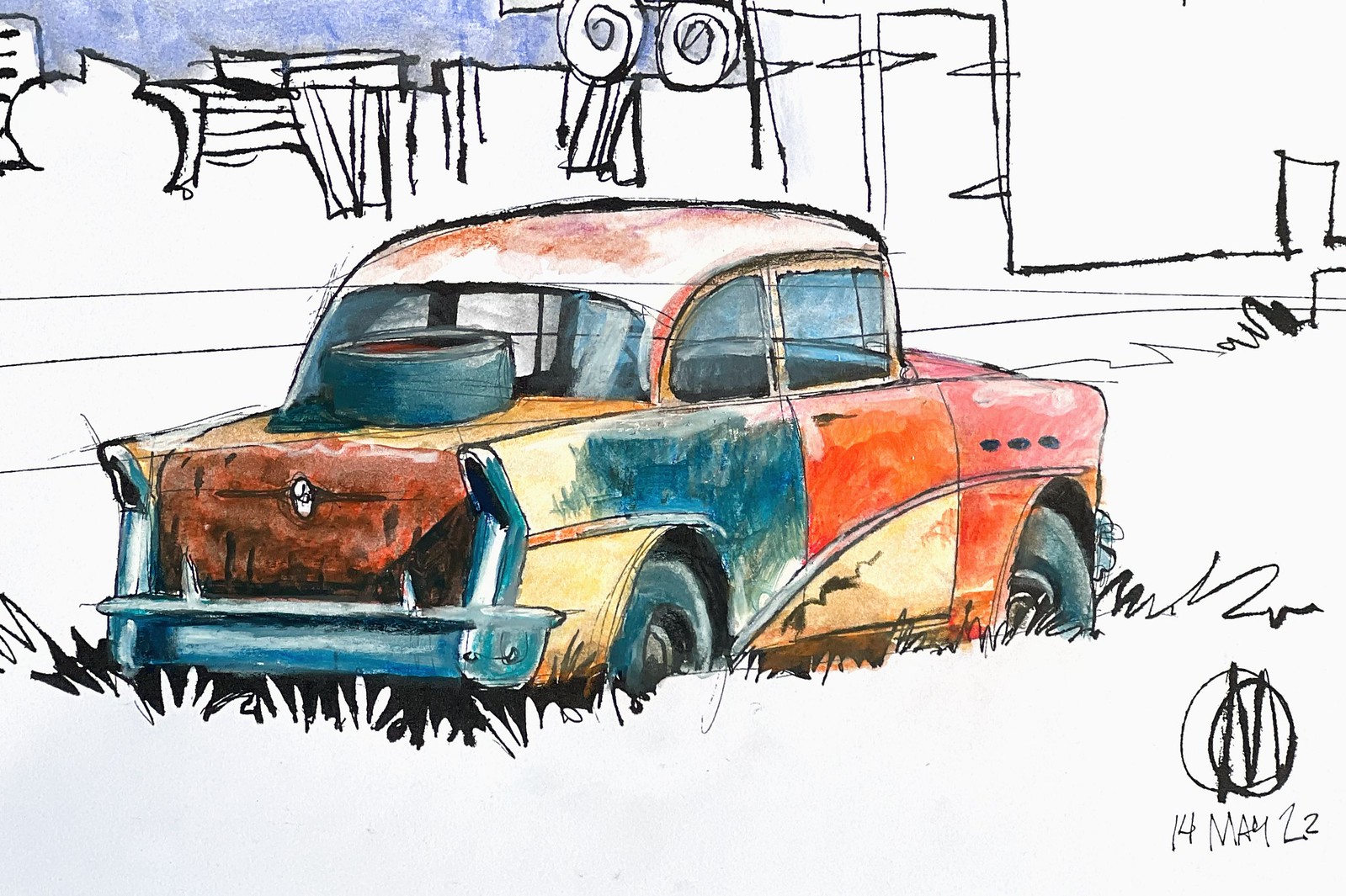The image is a detailed pen and ink drawing on white paper, depicting an old, broken-down car from the 1950s or early 60s, reminiscent of a Chevy, Ford, or Cadillac with rounded edges and fins. The car, stranded in a grassy meadow, exhibits a mishmash of colors—red, orange, blue, yellow, pink, and brown—indicating that different parts have been replaced over time. The trunk is heavily rusted and bears a single tire. The front right tire is flat, with tall grass encroaching around the vehicle's bottom. In the background, a cartoonish city skyline, drawn in black and white with simplistic, geometric shapes, stands under an azure sky. The grass and buildings lack color, emphasizing the car's vibrant patchwork. In the bottom right-hand corner, the artist's signature reads "OM" with overlapping circles, dated 14 May 22.